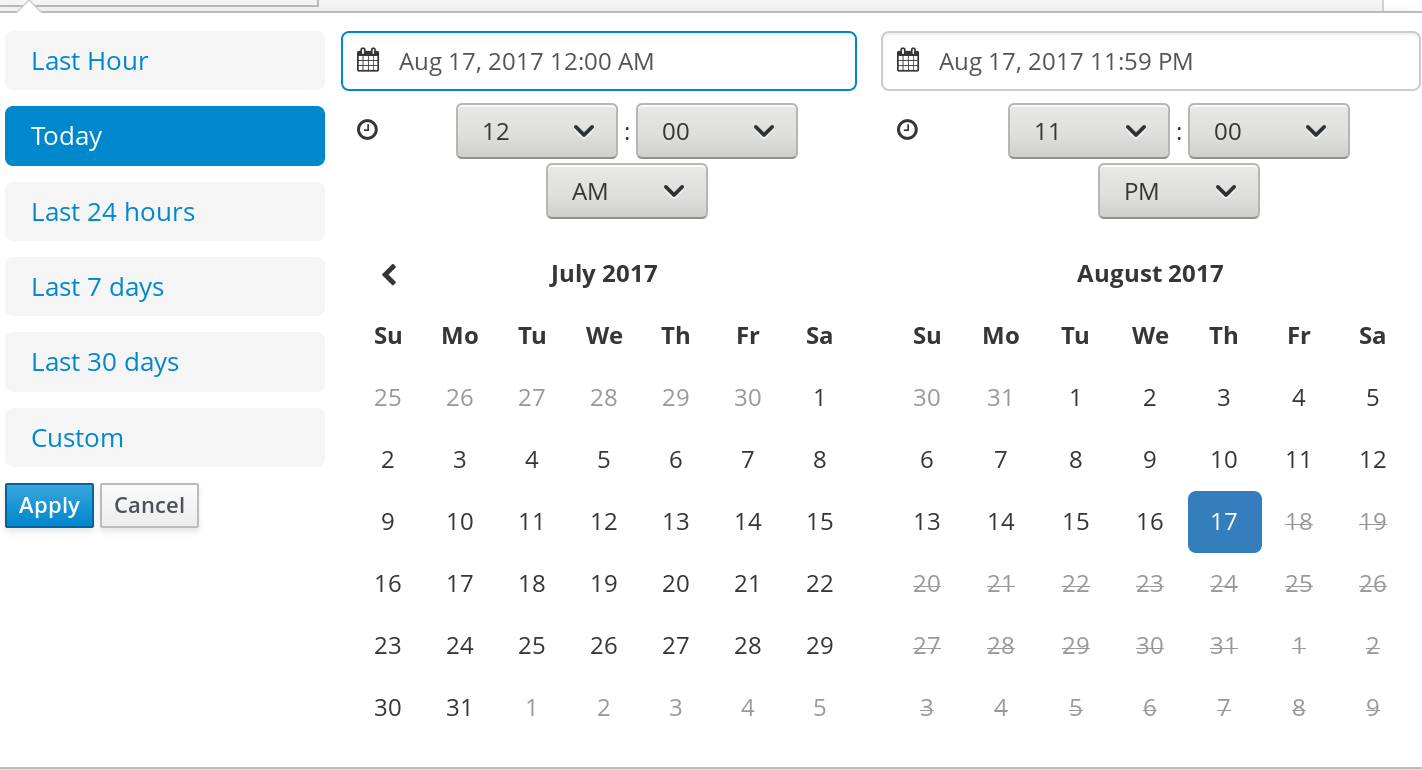This screenshot displays the calendar interface of the Microsoft Outlook or Microsoft 365 app on a PC laptop. The predominant background is white. On the left side, a vertical menu featuring six grey rectangular buttons is visible. These buttons are labeled in order: "Last Hour," "Today," "Last 24 Hours," "Last 7 Days," "Last 30 Days," and "Custom." The "Today" button, second from the top, is highlighted in cerulean blue with white text, contrasting the cerulean text of the other buttons. Below this main menu, there are two smaller buttons labeled "Apply" and "Cancel." To the right of the menu buttons, the interface displays two calendar pages showing July 2017 and August 2017. Dates past have greyed-out numbers and are struck through. At the top of the screenshot, a time span bar reads "August 17, 2017, 12 AM to August 17, 2017, 11:59 PM." Beneath this bar are grey controls for adjusting the date and time.